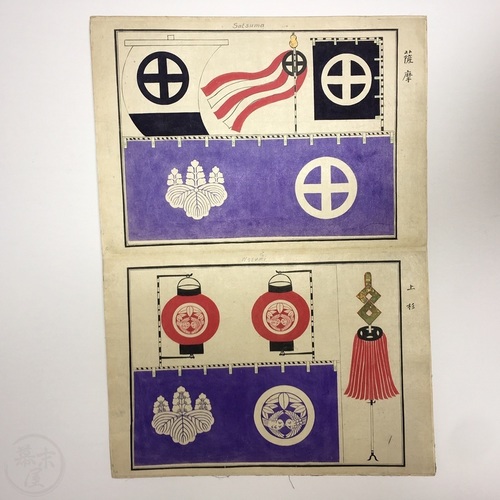The image depicts an old, yellowing piece of paper, possibly a poster or an open book, showcasing a variety of symbols and images. Central to the imagery is a repeated emblem—a circle with a symmetrical cross inside, symbolizing something unclear but consistently featured throughout the composition. 

In the top half of the image, this emblem appears in black against a white sail in the top-left corner. Adjacent to this, the same emblem is seen on a red and white striped flag, fluttering on a flagpole. Moreover, the emblem is displayed on a stationary flagpole in a black square on the top-right corner, creating a visual rhythm across the upper section. Flanking these elements are two blue bars with crenellations, as if depicting the top of a building. Each blue bar is adorned with a floral crest and the repeated emblem with three fronds and three stalks of plants.

The bottom half of the poster transitions into a more complex and densely packed area, featuring mandala-like symmetrical circles, though not actual mandalas, which are hard to describe. Among these are two red lanterns, each decorated with white crests, and a pole adorned with a red skirt and a metallic ornament at its top. 

Overall, the piece combines historical motifs and geometric symbols with intricate decorative elements, suggesting a blend of ceremonial and architectural significance.